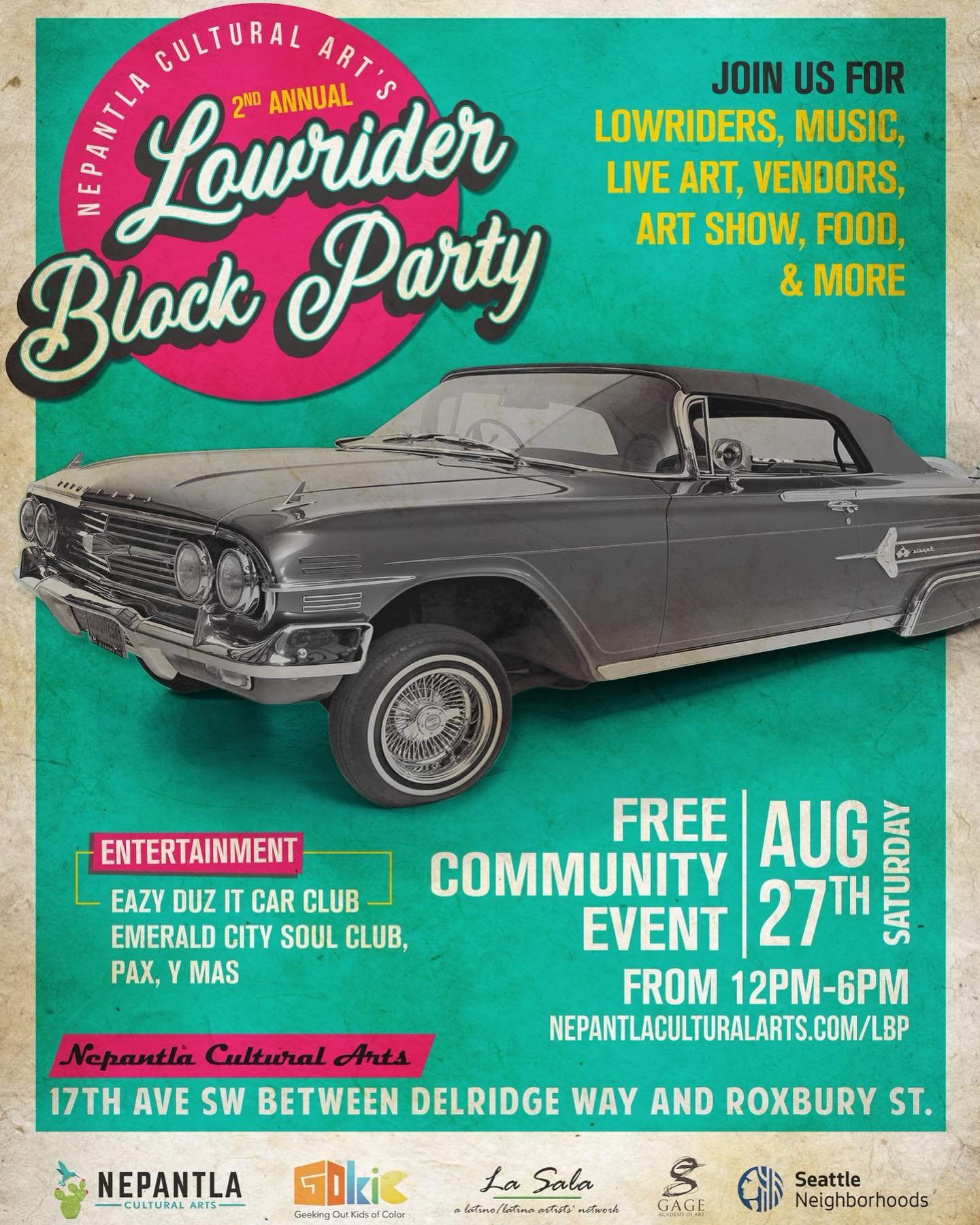The image is a poster promoting the Nepantla Cultural Arts Second Annual Lowrider Block Party. The poster has a distinctive retro look, with a light-colored, aged border featuring brown spots. In the top left corner, there's a lavender circle with "Nepantla Cultural Arts Second Annual Lowrider Block Party" written in white. The top right corner invites attendees to "Join us for Lowriders, Music, Live Art, Vendors, Art Show, Food, and More" in a mix of black and yellow text. The central image is a striking black-and-white photo of a lowrider car with its back end almost touching the ground and the front end significantly higher. Below the car image, the text announces a "Free Community Event," listing the date and time as "August 27th, Saturday from 12 p.m. to 6 p.m." and provides the website "nepetlaculturalarts.com/lbp." The poster is set against a cyan rectangle background and also mentions entertainment from "Easy Does It Car Club, Emerald City Soul Club, Pax Imas," along with a list of sponsors and the event's address at the bottom.